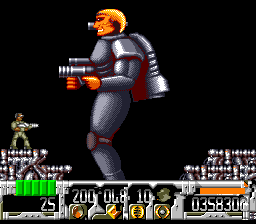The image features a video game character set against a pitch-black background. The character, who has distinct orange skin and shallow, possibly spiky, hair, is adorned in a blue outfit. Clutched in his hand is a futuristic-looking gun, suggesting a potential for combat or action scenarios within the game. Strapped to his back is a jetpack, indicating that the character may have the ability to fly or make high jumps.

In the foreground, positioned on a ledge, stands a smaller character—possibly an ally or another game element—also brandishing a large gun. This tiny figure adds a layer of complexity to the scene, hinting at interactive or strategic gameplay elements. 

In the bottom right corner of the image, a score display can be seen, highlighting the player's progress or achievements. On the left side, a series of green rectangles likely represent the character's health or life gauge, providing crucial information for the player to manage their character's vitality throughout the game.